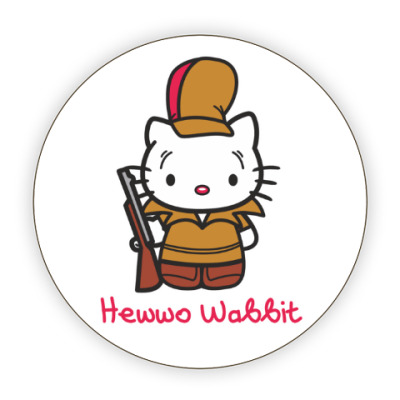The circular image features a detailed drawing of the beloved character, Hello Kitty, dressed as Elmer Fudd from Looney Tunes. Encircled by a thin brown or possibly black border, the central background is white, setting off the character prominently. Hello Kitty, depicted in her classic white form, stands upright, donning a distinctive brown, conductor-style hunting hat with a red stripe. She is attired in a matching brown shirt and darker brown pants, though her feet are not visible. Her ensemble is completed with a brown rifle, featuring a wooden stock and a gray barrel, held in her paws. Notably, Hello Kitty’s facial features include a red or possibly pink nose, black eyes, and whiskers. Below the character, "Hello Wabbit" is playfully written in red text mimicking a child’s speech, with "H-E-W-W-O-W-A-B-B-I-T" in a mix of capital and lowercase letters. This image cleverly parodies Hello Kitty as Elmer Fudd, creating a unique and whimsical visual.